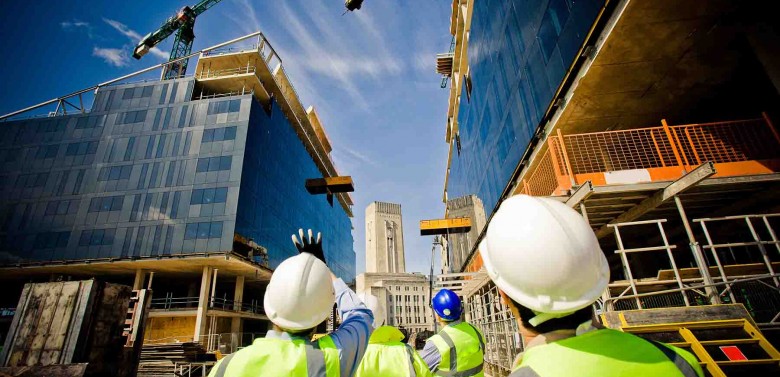In the bustling city backdrop, the image depicts an active construction site where four men, donned in safety gear, are engrossed in their tasks. Three wear white hard hats, while one sports a blue hard hat; all are clad in bright green safety vests that stand out vividly against the urban landscape. The workers' attention is riveted upwards towards a towering crane that looms in the sky, its presence marked against the blue sky with streaks of lined clouds. The men are positioned between two partially constructed buildings featuring shiny gray surfaces interspersed with exposed wooden beams and planks, indicating their yet-to-be-completed state. One of the workers, distinguished by his raised hand, appears to be signaling the crane operator, perhaps guiding its movements. Nestled amongst this construction site is a fully completed, cream-colored building, providing a stark contrast to the work-in-progress structures. Additional details capture the environment's complexity: a lower central building, an orange-fenced area beneath a dark brown structure on the right, and scattered scaffolding indicating ongoing activity. Together, these elements capture a moment of precision and coordination in the heart of city construction.